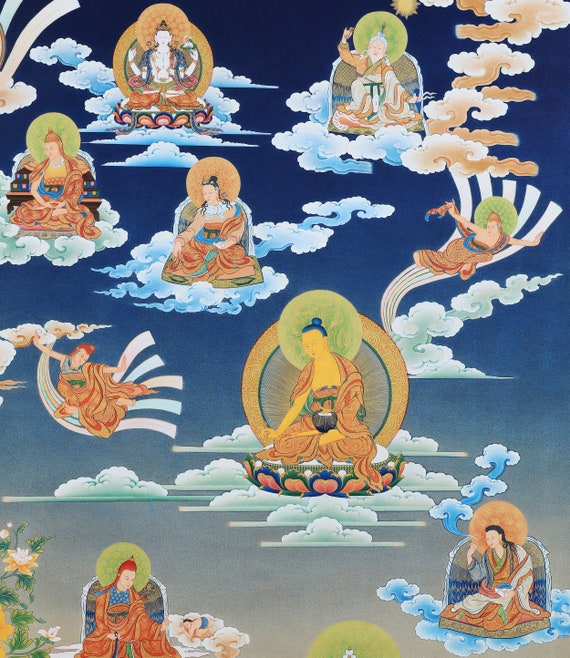This digital artwork features an intricately designed print depicting various Indian gods, each styled with an Asian influence. Set against a blue background, the figures are scattered across white, floating clouds, exuding a serene and spiritual ambiance. There are approximately nine deities, all characterized by their robes and distinct hairstyles, many with buns. Each figure appears to be deeply engaged in different activities, such as preparing offerings or praying, often looking down at something in their laps. Behind their heads, circular auras signify their divine status. The palette of the artwork includes tans, whites, greens, blues, and hints of red, contributing to its vibrant yet harmonious appearance. This stylized print is versatile and could be used on various products like wrapping paper, material, t-shirts, or posters, making it a suitable decorative piece for those interested in religious or cultural art, similar to what might be found on platforms like Etsy.